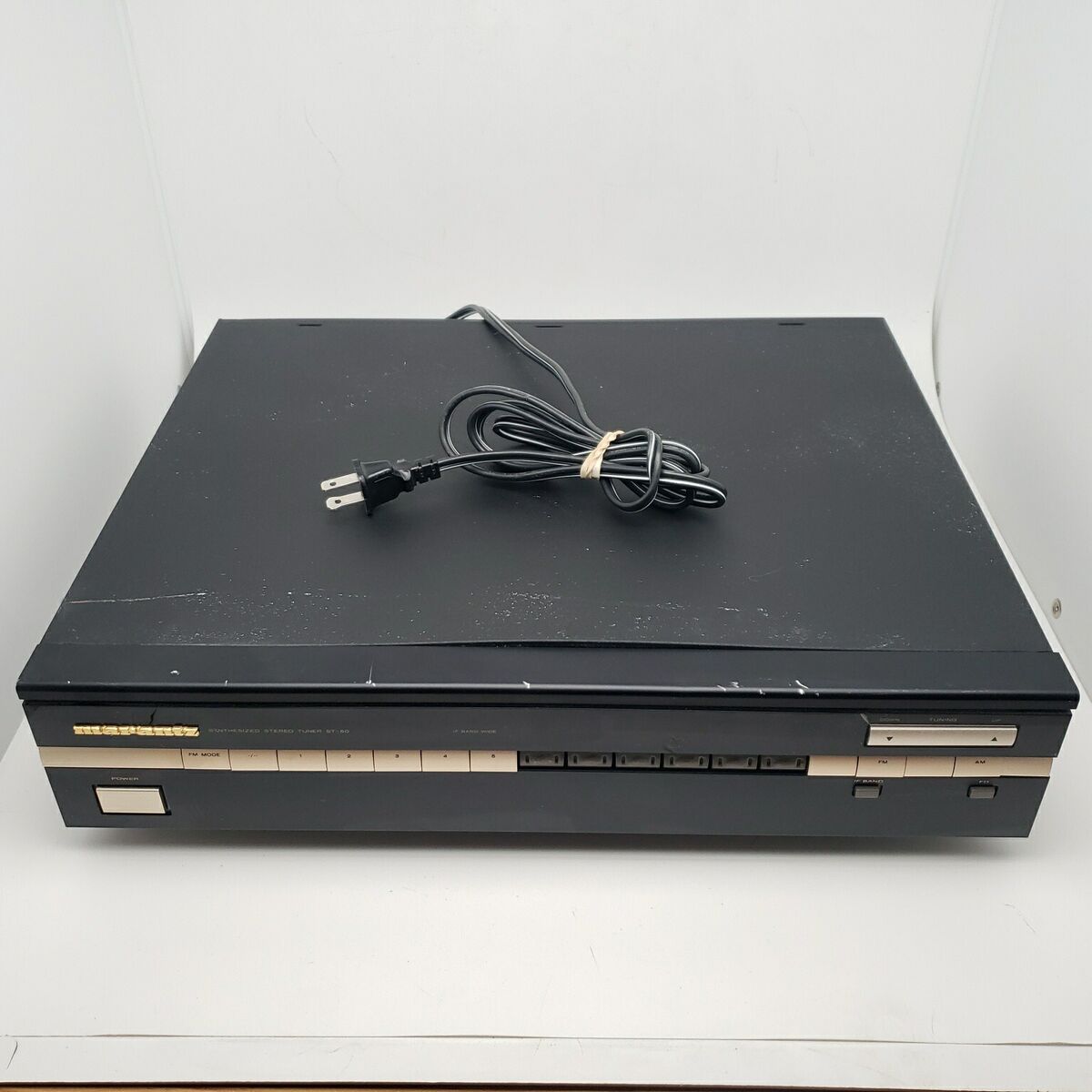This photograph showcases a piece of vintage technical equipment, likely an early disc player, set against a very light gray background. The device itself, characterized by its metal construction, presents as a horizontal, flat black rectangle, approximately 8-9 inches square. Its front face features a row of gold or light brown push buttons, though the specific labels on these buttons remain indistinguishable. An additional gold horizontal rectangle, possibly an input slot, is situated on the upper right-hand side, suggesting functionality related to media insertion. The unit seems well-used, displaying evident nicks, scrapes, and scratches on its top and faceplate, indicating frequent movement over time. A neatly wrapped black plug-in cord, secured with a beige tie, extends from the device. Despite its worn condition and uncertain operational status, this piece encapsulates a slice of technological history.